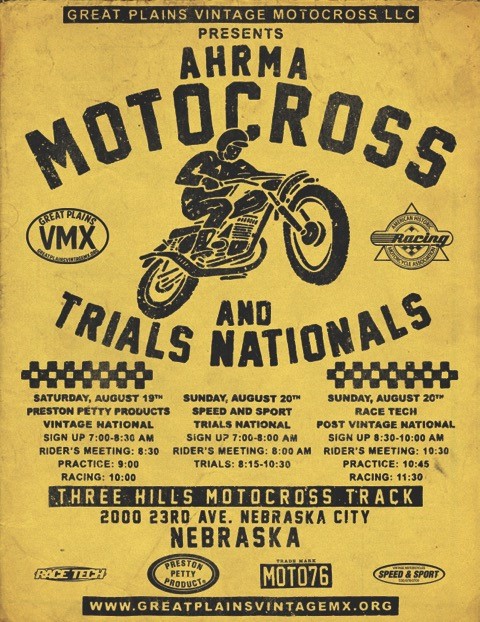This vertically rectangular poster, with a yellow to yellowish-orange background and black text, advertises the Desert Plains Vintage Motocross LLC's event, specifically the AHRMA Motocross and Trials Nationals. At the top, a black banner prominently displays "Desert Plains Vintage Motocross LLC presents AHRMA Motocross and Trials Nationals." Below this header section, there are two sponsor logos flanking an illustrated, blacked-out image of a man riding a motocross bike. On the left, an oval logo reads "Great Plains VMX," while on the right, a triangle with a circle inside it bears the word "Racing."

The poster includes detailed event information. For Saturday, August 19th, featuring the Preston Petty Products Vintage Nationals, sign-up occurs from 7 to 8:30 AM, followed by a Riders Meeting at 8:30 AM, Practice at 9 AM, and Racing at 10 AM. Sunday's lineup for August 20th includes the Speed and Sport Trials Nationals, with sign-up from 7 to 8 AM, a Riders Meeting at 8 AM, and Trials events at 8:15 and 10:30 AM. Additionally, on Sunday, the Race Tech Post Vintage Nationals has sign-up from 8:30 to 10 AM, a Riders Meeting at 10:30 AM, Practice at 10:45 AM, and Racing at 11:30 AM.

At the bottom, the poster provides the location information: Three Hills Motocross Track, 2023rd Avenue, Nebraska City, Nebraska, and the website www.greatplainsvintagemx.org. Additional sponsor logos are positioned near the bottom, enhancing the informative yet straightforward design of the poster.